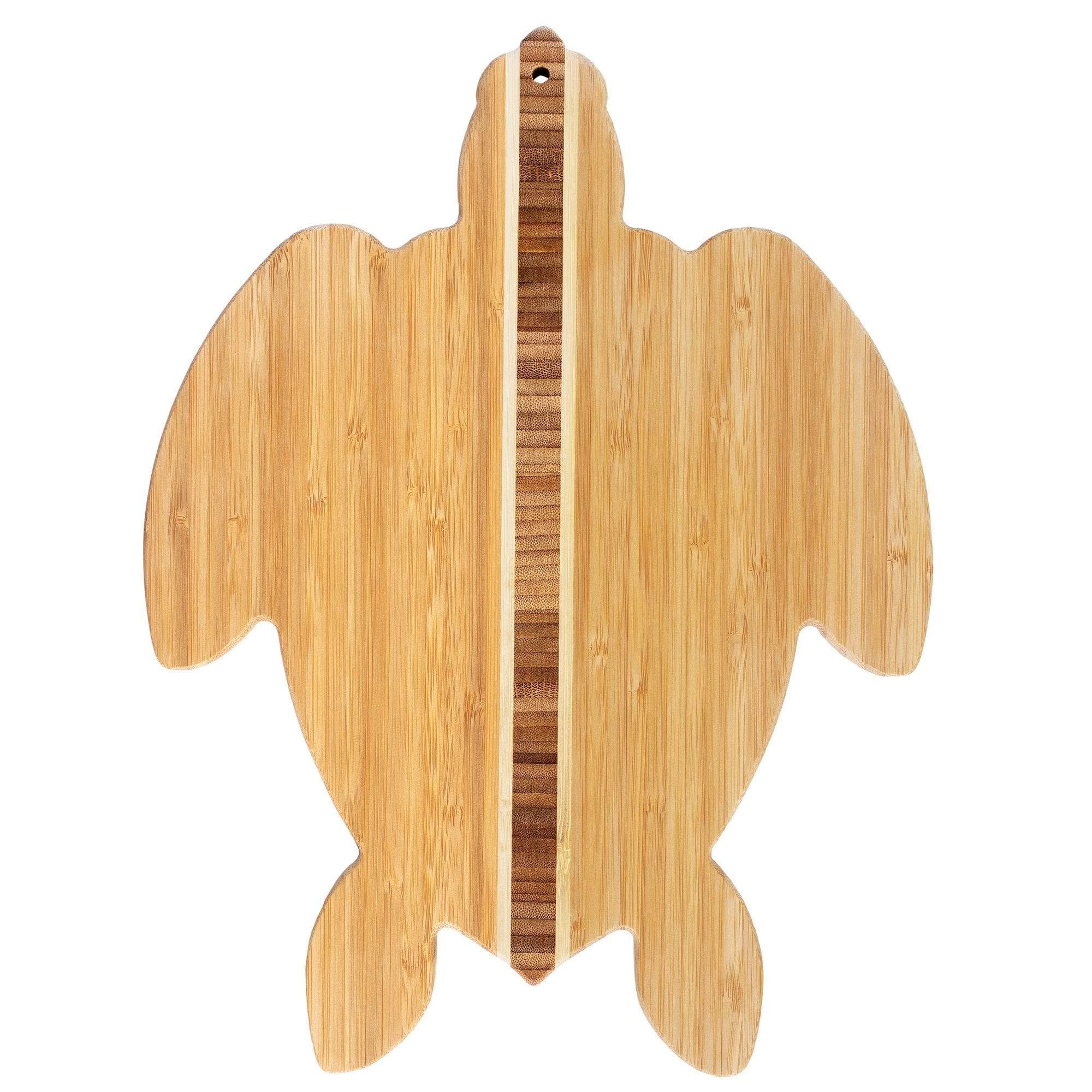This image captures a uniquely designed cutting board shaped like a sea turtle, set against a plain white background. The board is crafted from multiple types of wood, featuring a main body of light beige wood, possibly bamboo, with a pronounced vertical grain running top to bottom. The turtle-shaped board includes distinct anatomical details such as long front flippers, a smallish head at the top, and two small, circular back flippers at the bottom.

Central to the design is a striking horizontal strip of darker wood, standing in contrast to the surrounding lighter wood and lending a sense of depth and texture to the piece. This central strip is accented with very pale wood strips on either side, creating a visually appealing contrast. The darker strip appears to be composed of multiple small pieces of wood, each oriented horizontally, differing significantly in grain direction from the rest of the board.

A small hole drilled at the top, positioned where the turtle’s eyes would be, serves as a practical feature for hanging the cutting board. This combination of functionality and artistry makes the turtle-shaped cutting board both a useful kitchen tool and a potential decorative piece.